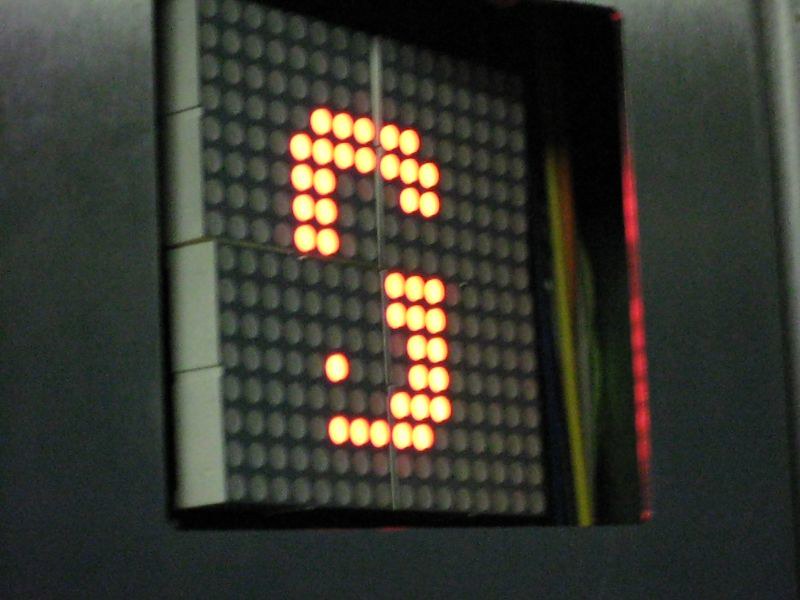This color photograph appears to be a close-up of an outdoor digital sign, potentially a clock or a display unit. The frame of the sign is dark gray, enclosing a square section that functions as the display area. Within this square, there are segments resembling blocks with numerous small dots, some of which are illuminated in a bright reddish-yellow hue. These illuminated dots form a partially lit character that could either be the letter "G" or the number "6," though the incomplete lighting makes it hard to discern definitively. Additionally, a few visible cords can be seen running down along the right side of the digital display, adding to the intricate detail of the scene.